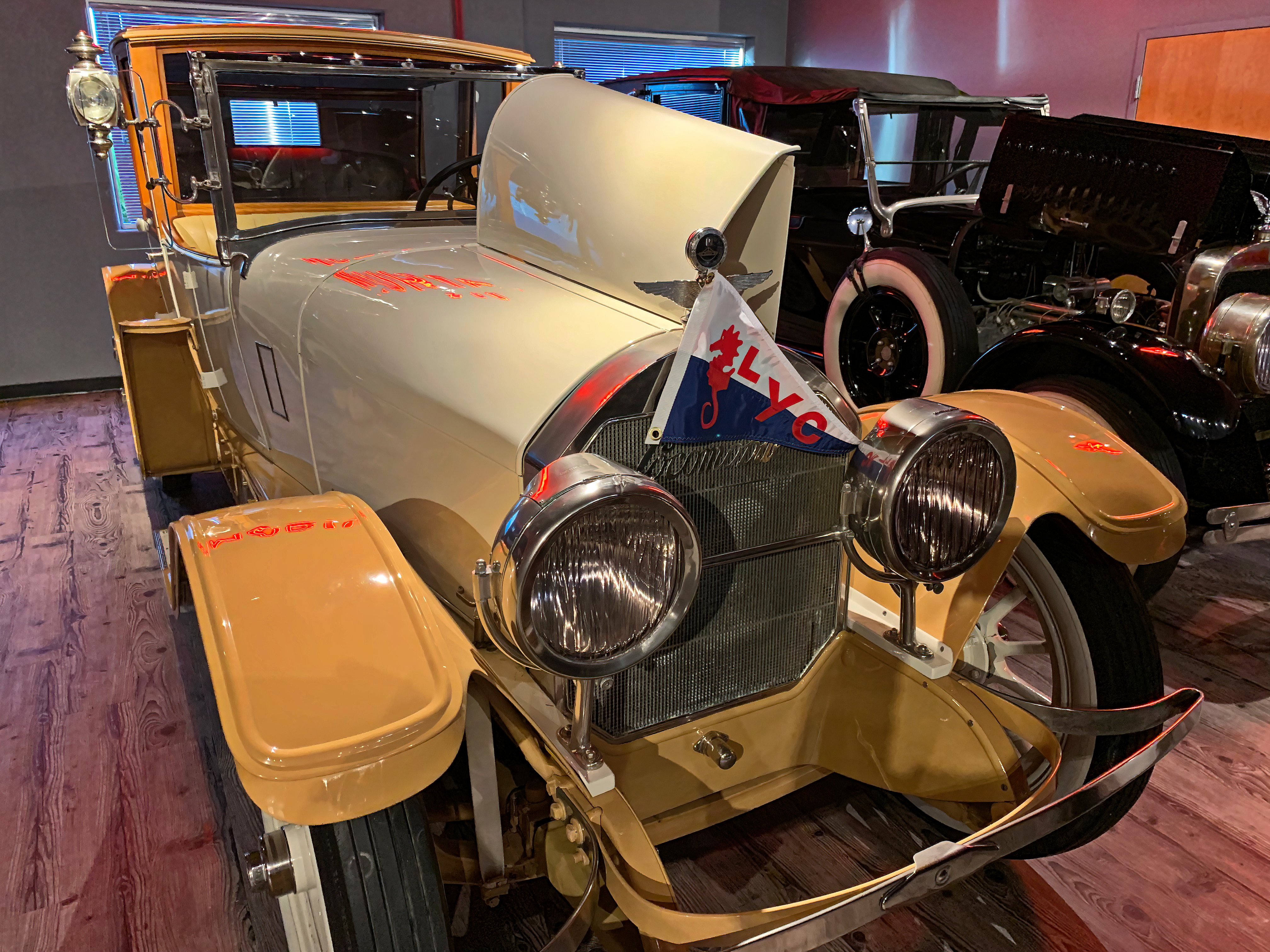The image captures a scene from a car show held indoors, potentially in a museum setting. The setup resembles a house or a small room with wood-look flooring and walls featuring two windows, offering a cozy yet unusual display environment. The primary focus is on a vintage yellow car from the early 1900s, adorned with a cream and white hood, and remarkable for its yellow fenders covering the tires. This car has its hood open on the right side, revealing shiny internals, with a silver grille and silver headlights enhancing its classic aesthetic. Affixed to this car is a triangular flag, blue at the bottom and white at the top, showcasing a red seahorse and the letters "LYC." Alongside this centerpiece are other antique vehicles, including a black car with white details and a chrome grille, which also has its hood opened. The absence of any identifying marks or people further suggests a meticulously curated and quiet exhibition space, perhaps resembling a bedroom without furniture, underscored by exhibition-style lighting that emphasizes the historical significance and beauty of these vintage automobiles.